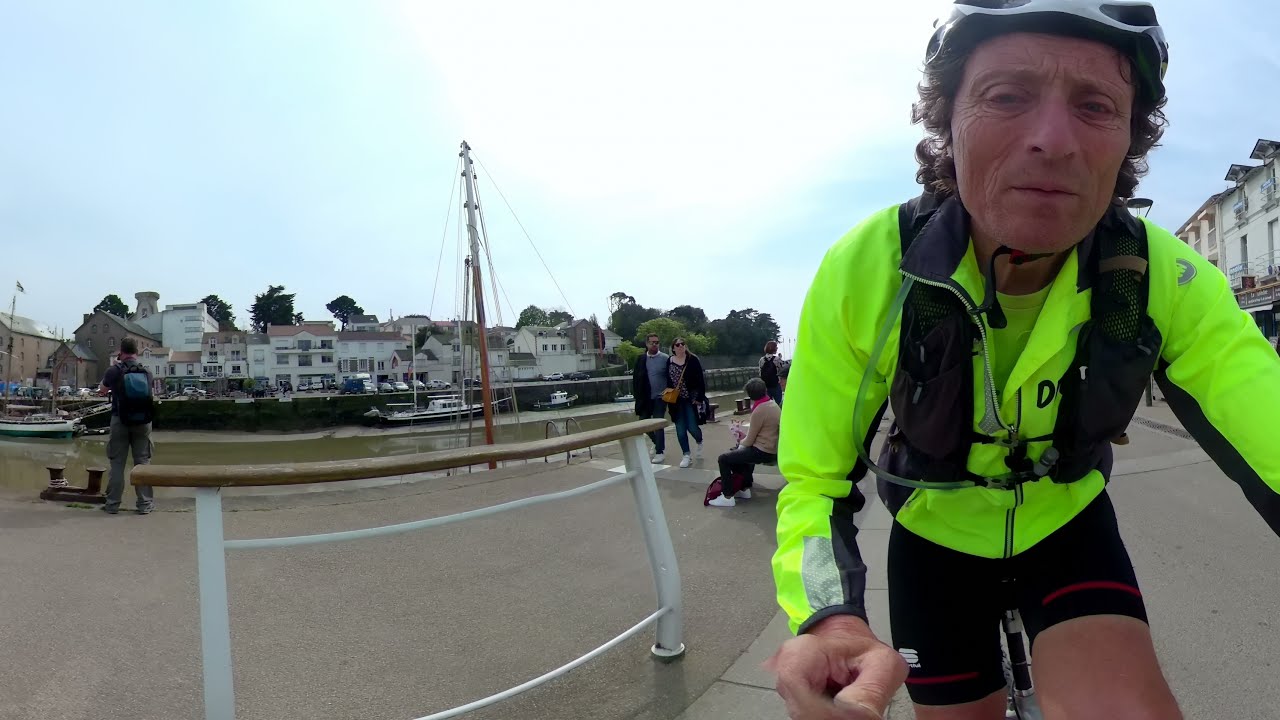A vivid outdoor scene captures a bicyclist from a handlebar-mounted camera. Positioned on the right side of the image, the cyclist is attired in black spandex shorts and a bright neon yellow jacket with black detailing, complemented by a white and black helmet. The cyclist faces the camera, with a background featuring rows of closely packed white houses and a serene bay area dotted with boats. To the left, three boats are tied off to a concrete dock, where people are leisurely walking and sitting. A couple in black clothing strolls by, while another duo sits on a concrete bench. There's a man standing near a metal concrete anchor, gazing at the water. The sun is shining brightly, with a clear sky adding to the picturesque quality of the neighborhood and the water, which is framed by homes and boats.